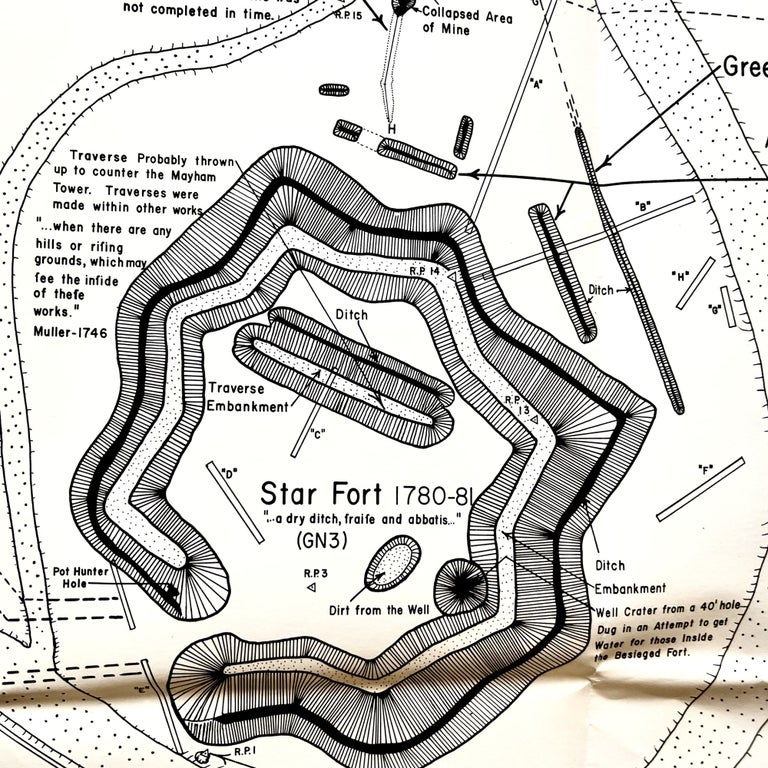This image is a detailed black and white photograph of an aged topographical map, showcasing the schematics of a complex structure known as a Star Fort. The fort itself is depicted in an octagonal shape and is surrounded by various intricate features and descriptive labels. At the top of the map, a portion is marked "collapsed mine area," while the central part of the image illustrates an embankment within a dry ditch, creating a loop-like irrigation system. The upper left corner contains a detailed quote about traverses constructed to counter the Mayhem Tower, noting their utility in rough terrains. The bottom right corner features a note about a "Well crater from a 40-foot hole" dug for water. The map, drawn in black ink on creamy, yellowish, aged paper, includes additional labeled elements such as "ditch", "embankment", and "Pot Hunter Hole," accompanied by smaller sketches that surround the main structure. The intricate network of features and annotated notes reflect an architectural design and strategic planning context.